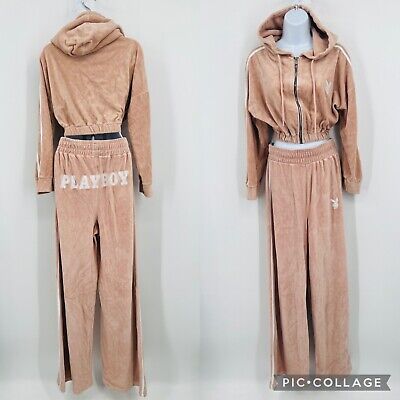This is a color photograph displaying a dusty pink leisure wear set, consisting of a hoodie and matching sweatpants, presented in two separate images. On the left side, we see the back view of the outfit, which is hanging on a hanger. The hoodie features a hood hanging down and long sleeves, while the sweatpants are detailed with a drawstring waist and slits running up the sides. Notably, "Playboy" is printed in white letters across the buttocks area of the pants. 

The right side of the photograph shows the front view of the ensemble on a white, headless mannequin. The hoodie displays a black zipper running down the middle, with drawstrings coming down from the hood, which is pulled over the top part of the mannequin's neck. Additionally, a Playboy Bunny logo is positioned over the left breast and on the upper thigh area of the sweatpants. The image is framed with the bottom right corner displaying the words "PIC collage," suggesting it might be part of a social media post or a catalog.